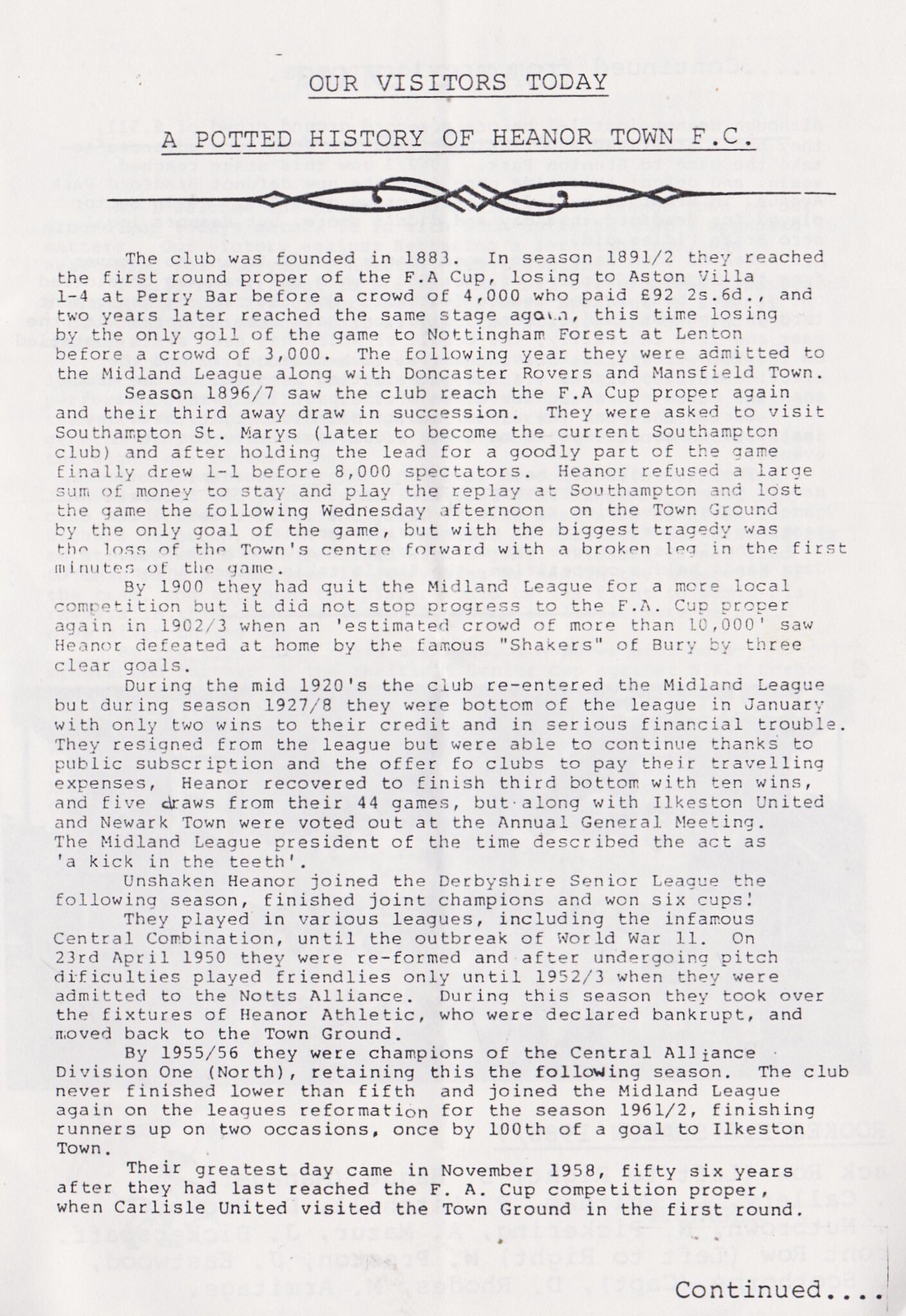The image displays an aged white piece of paper featuring a memo titled "Our Visitors Today" in all capital letters, underlined by a decorative line. Below this heading, the title "A Potted History of Heanertown F.C." (Heanor, H-E-A-N-O-R) is prominently displayed. The page includes a detailed history, mentioning that the club was founded in 1883. It highlights a significant event from the 1891-2 season when they reached the first round proper of the FA Cup, losing 1-4 to Aston Villa at Perry Bar before a crowd of 4,000 who paid £92. Two years later, Heanertown F.C. reached the same stage again, losing before a crowd of 3,000. The following year, the club was admitted to the Midland League along with Doncaster Rovers and Mansfield Town. The text comprises eight paragraphs, detailing these historical highlights, and at the bottom, it indicates "continued."

The decorative line beneath the titles starts as a straight line, transitioning into an open diamond, followed by a long oval shape, and then curving upward and downward, forming a unique separator before the historical content begins.